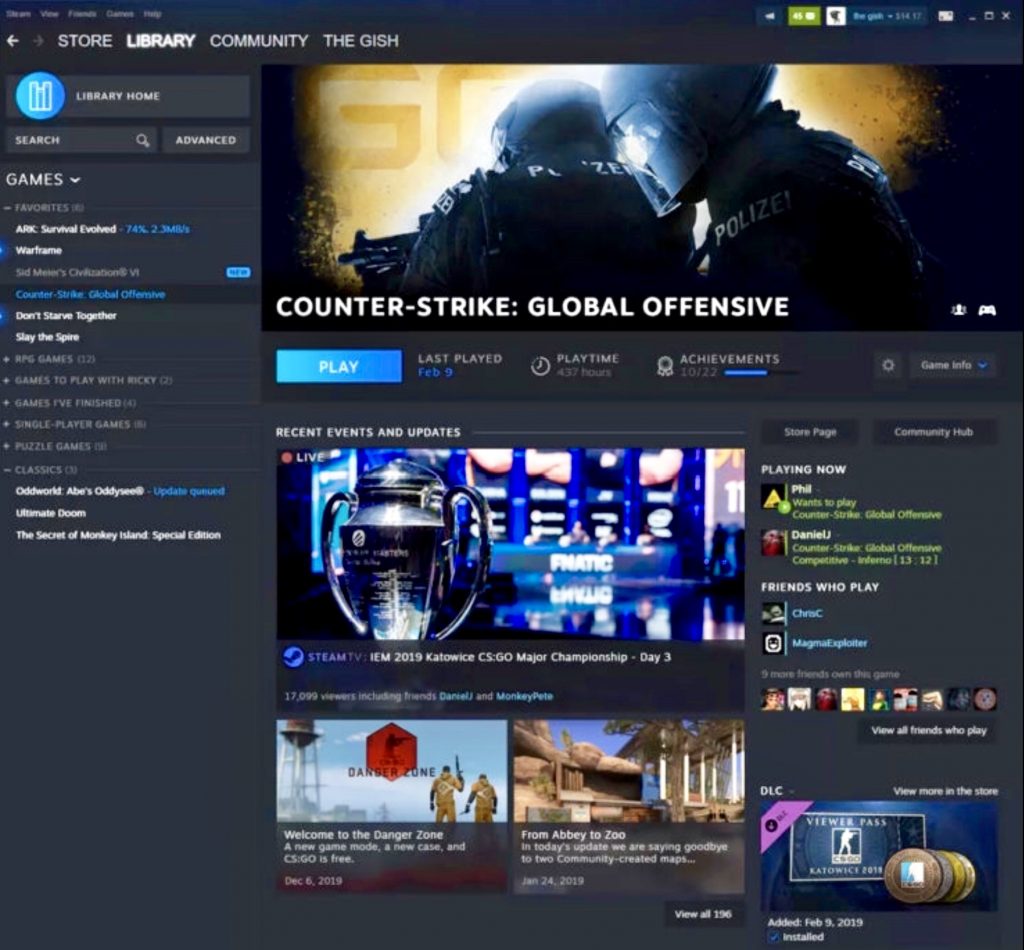**Detailed Caption for Image:**

The image depicts a personalized gaming interface on a library's web page, showcasing a film related to the game Counter-Strike Global Offensive. The striking black background provides a stark contrast to the typical library homepage design, making this display unique. At the very top, key navigational elements are highlighted in white: the options for 'Store,' 'Library,' 'Community,' and 'About.' Additionally, a small blue circle featuring three books serves as the library's icon.

Above the search bar, represented by a magnifying glass icon, users can search for games, advanced options, and favorites. This specific user has favorites listed such as Ark: Survival Evolved and Warframe. Notably, other games, including Counter-Strike Global Offensive, Don't Starve Together, Slay the Spire, and various genres like RPG games and single-player classics, are organized on the left-hand side. Categories include 'Games to Play with Friends,' 'Games I Finished,' 'Single-player Games,' 'Puzzle Games,' and 'Classics,' with notable titles like Oddworld, Ultimate Doom, and The Secret of Monkey Island: Special Edition.

The central part of the image showcases the promotional banner for Counter-Strike Global Offensive, featuring heavily armed characters in combat gear. The foreground figure is brandishing a rifle, while a background figure supports them. This section also includes highlights such as 'Playing Now,' 'Recent Events and Updates,' and specific game modes like 'Welcome to the Danger Zone' from Abbey to Zoo.

Furthermore, the interface details the user's friends who play similar games, along with a 'Viewers Pass' from DLC, added on February 9, 2019. Prominently, the word 'play' is highlighted in blue, showing the last played date (February 9th), total playtime (437 hours), and achievements (10 out of 22), with a progress bar visually representing the accomplishments. This comprehensive layout illustrates how the user engages with the library’s extensive gaming collection via their customized webpage.